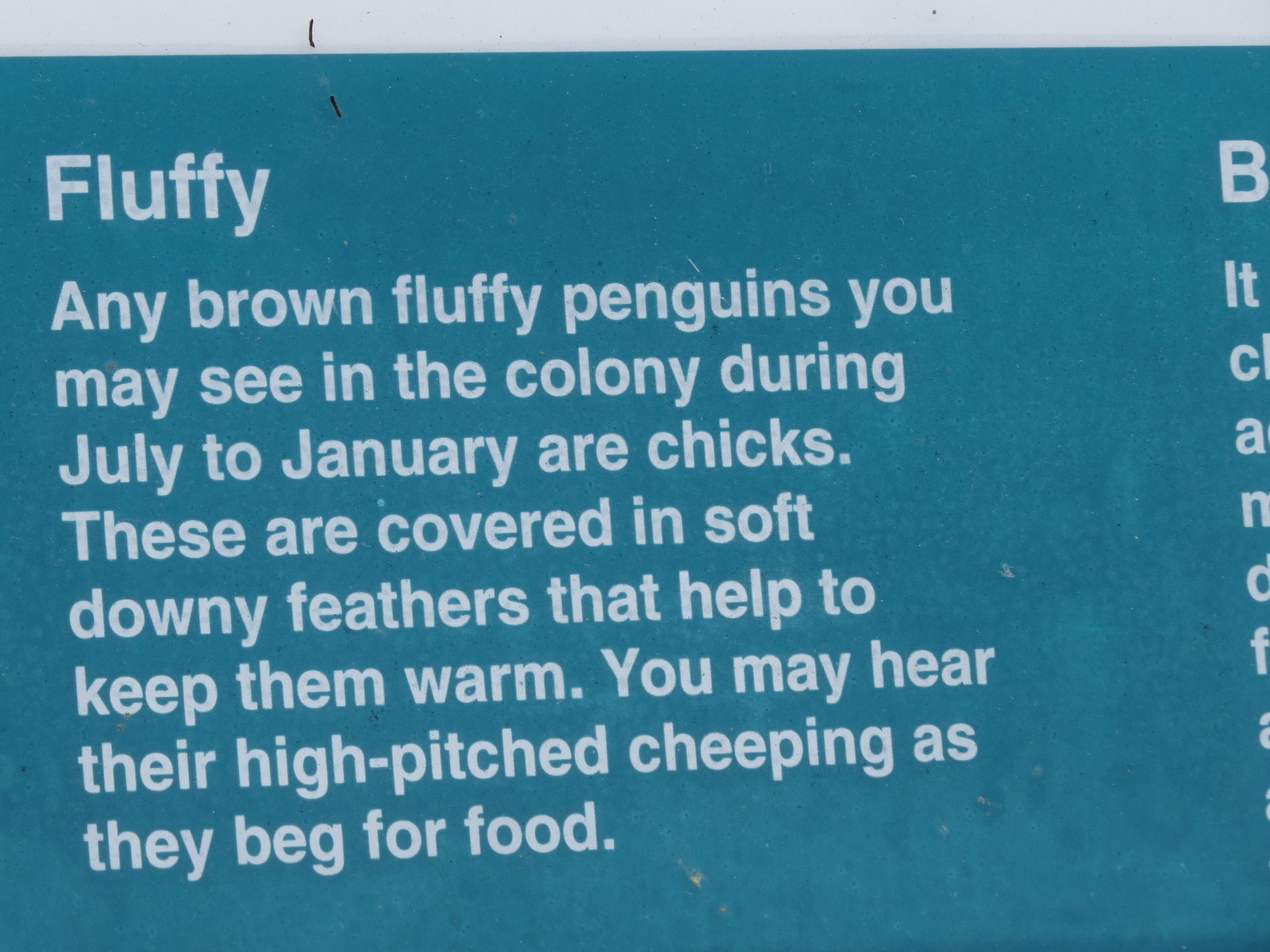The image is a horizontal, rectangular piece with a light gray border that narrows from the upper left to the lower right, suggesting the photograph is slightly tilted. The background is a dusty bluish-green color with white text. At the top left, in bold letters, the title "FLUFFY" is prominently displayed. Below the title, the text reads: "Any brown fluffy penguins you may see in the colony during July to January are chicks. These are covered in soft downy feathers that help to keep them warm. You may hear their high-pitched cheeping as they beg for food." On the right-hand side, partially cut-off white text forms incomplete words due to the tilted angle. The overall aesthetic suggests an informative display about penguin chicks, emphasizing their appearance, behavior, and distinctive sounds. The photo appears pinned to a backboard with a black pin.